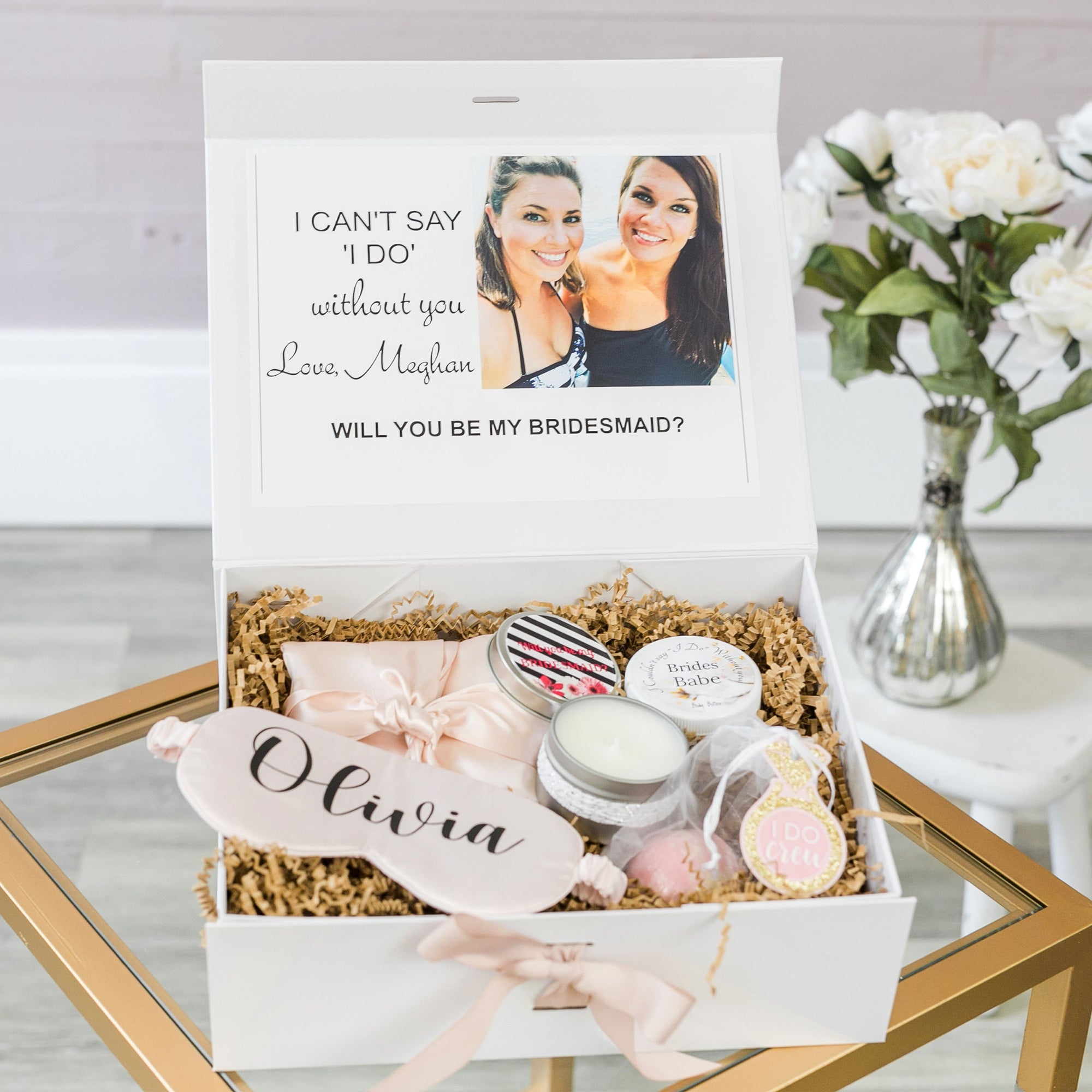This photograph captures a beautifully arranged bridesmaid gift box, prominently placed on a small glass table bordered with gold. The white box, elegantly tied with a pink bow at the front, is open, with its lid propped up against the back. The lid displays a heartfelt message on a card that reads, “I can’t say I do without you. Love, Megan,” alongside a photo of two women and the question, “Will you be my bridesmaid?” in bold black letters.

Inside, the box is lined with gold-colored ribbon and filled with delightful items: small white jars likely containing cosmetics, a plastic-wrapped item at the bottom right, and a sleep mask bearing the name "Olivia" on the bottom left, suggesting the recipient's name. In the background, to the right, sits a vase filled with elegant white roses, completing the scene with a touch of sophistication and warmth.